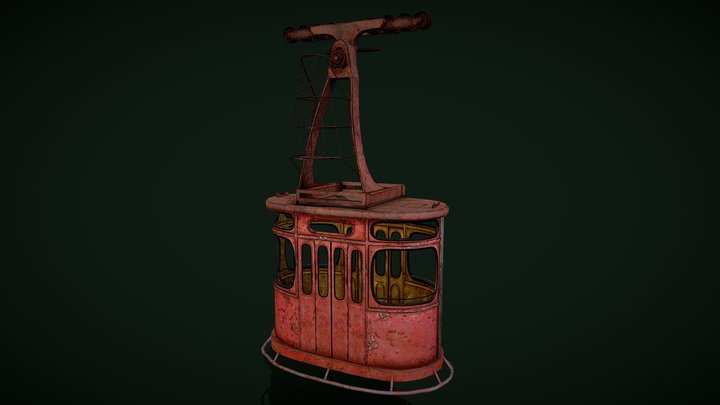The image depicts a detailed 3D rendering or illustration of a weathered, vintage, red gondola-like trolley car designed to travel on a zipline or cable. The car features a rusted, light red exterior, reflecting its worn-down condition. It is positioned against a dark, black background with hints of a greenish gradient in the corners. The car’s structure includes rounded corners and a large, squarish observation area with large, open window holes, lacking glass. The interior is a light brown shade, visible through the openings, while the roof is topped with a distinct, triangular metallic post that supports a substantial T-bar, meant for attachment to the zipline cables. The base of the trolley car is supported by a prominent metal post with additional welded support structures.